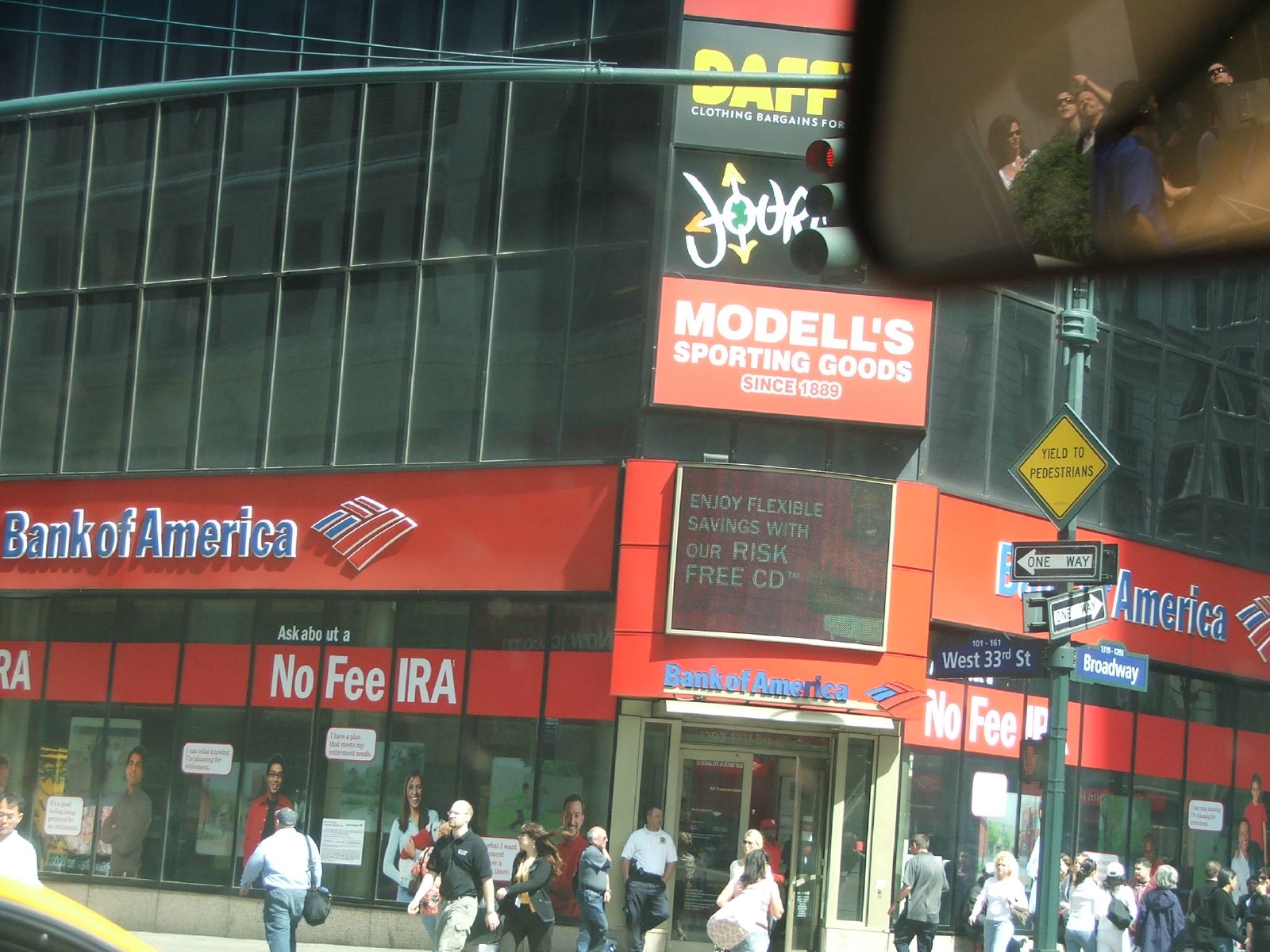This detailed color photograph captures a bustling city scene focusing on a commercial Bank of America building positioned at the intersection of West 33rd Street and Broadway. The building, predominantly black with accents of red, white, and blue from the Bank's branding, dominates the image. The Bank of America logo is prominently displayed on a red horizontal strip on both sides of the building corner. Promotional texts are displayed in green advertising a no-fee IRA. Above these, vertically aligned advertisements for Modell's Sporting Goods and Journeys add splashes of green, red, yellow, and black. A street signpost, grey and yellow, marks the intersection, reading "Yield to Pedestrians," "One Way," "West 33rd Street," and "Broadway." The lower eighth of the image presents a street view bustling with pedestrians wearing white and black attire. In the top right corner, a mirror – possibly from a motorbike – reflects additional street activity. The scene, with its intricate details and vibrant colors, portrays the essence of a busy urban environment.